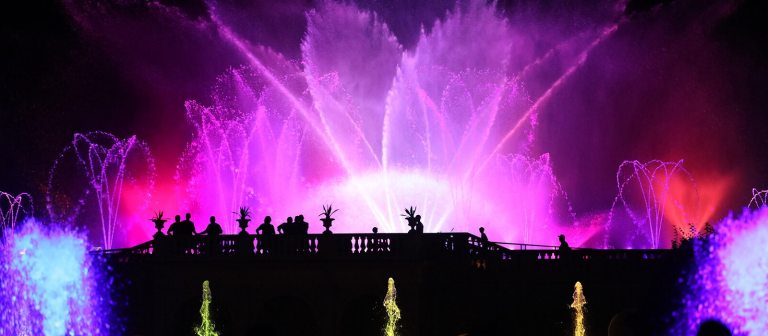The image captures a vibrant outdoor scene dominated by a stunning water show. Multiple fountains are shooting jets of water high into the air, illuminated by a captivating array of accent lights in shades of pink, purple, blue, and yellow. Prominently, on the bottom left, one fountain stands out with its deep purple hue, complemented by an intense electric blue nearby. Smaller yellow-lit fountains punctuate the middle, while the bottom right features another striking purple water jet. Silhouettes of people, rendered black against the backdrop due to the lighting, sit or stand on a platform that resembles a pier, observing the mesmerizing display. Enveloping the scene are pots with vibrant plants, adding a natural touch amid the high-energy spectacle. The sky above is a solid black canvas, enhancing the vivid colors of the water and the overall ethereal atmosphere of this dazzling nighttime show.